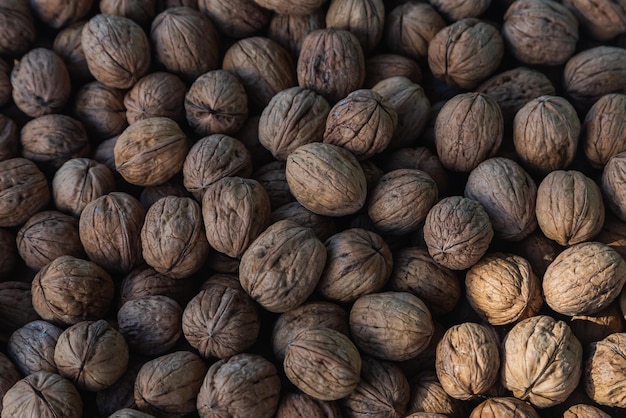The image depicts a large pile of walnuts taking up the entirety of the frame, extending from top to bottom and left to right. The walnuts, which are still within their shells, appear to be stacked fairly deep, with an intricately rough and wrinkly texture. The shells exhibit multiple cracks and ridge lines that run vertically from the base to the top. They vary in color from light brown to dark brown, and some even possess a purplish hue or a slightly greener shade. The image is layered with approximately a hundred walnuts, showing a gradient of shades influenced by lighting; the bottom right corner displays lighter and brighter walnuts due to sunlight, while the top left corner has darker walnuts. The majority of the walnuts share a central seam where they can typically be cracked open, with their surfaces marked by black ridges and occasional black dots.